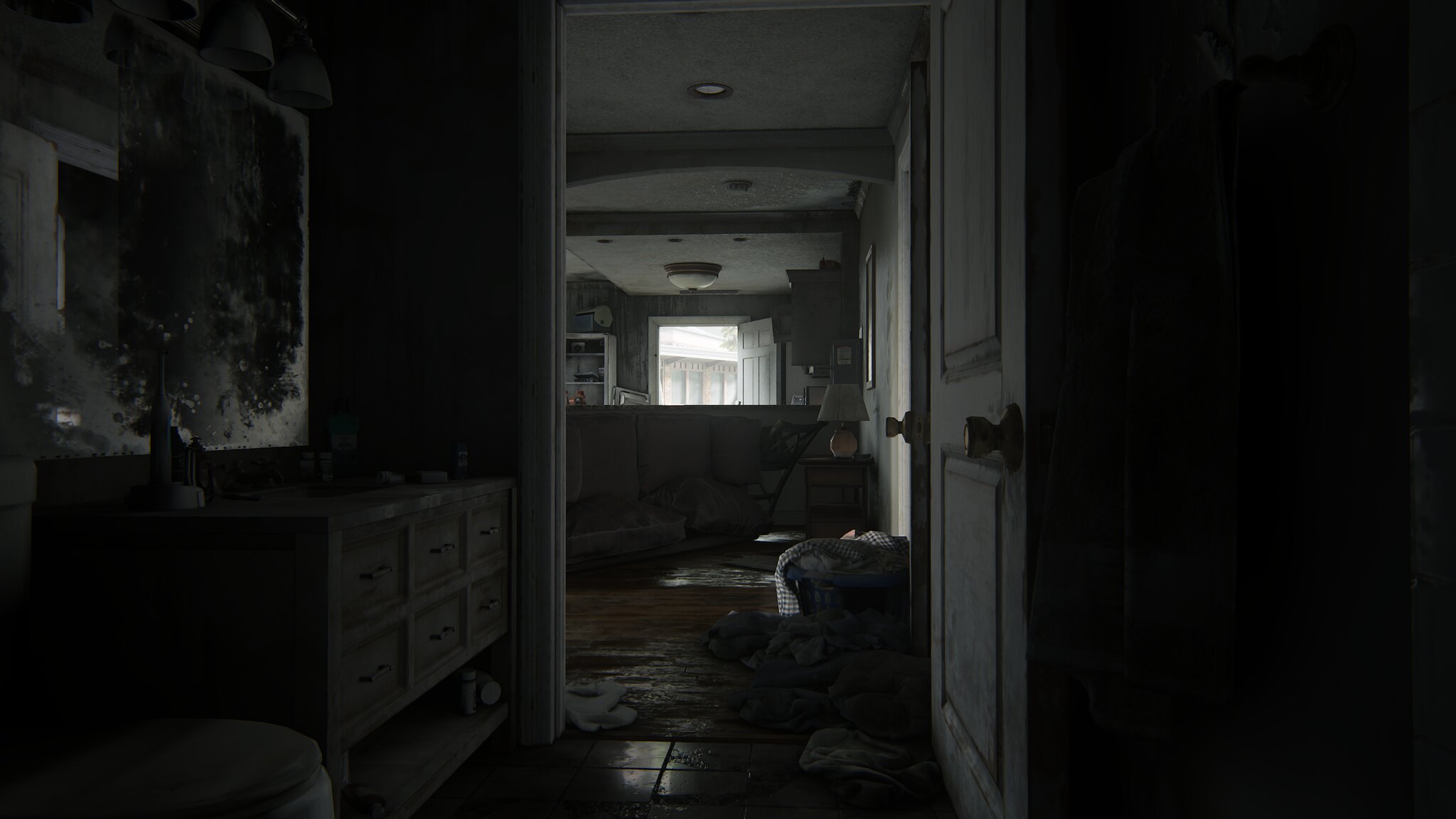This image captures a mysterious and dimly lit interior view, likely within a home. The perspective is from within a dark room, peering through an open door that swings to the right. To the left of this doorway stands a small dresser, which possibly holds a mirror above it, though the details are shrouded in shadows. This dresser may also be part of a vanity area in a bathroom. The adjoining room, also enveloped in darkness, features a small table lamp resting on a side table. In the background of this secondary room, a second door stands open, allowing a sliver of sunlight to pierce through, hinting at daylight beyond the confines of these shadowy interiors.